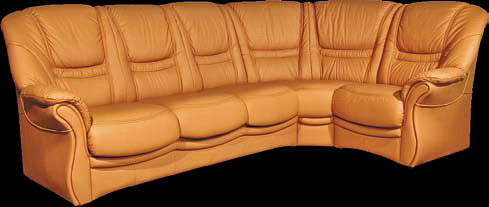The photograph features a large, wraparound couch set against a stark black background, likely intended for promotional or advertisement purposes. The couch, upholstered in a light pumpkin or tan-orange leather or faux leather, includes five seats: three aligned in a straight row on the left, a curved middle section that turns to the right, and two additional seats extending perpendicularly from the middle. The couch is designed with one armrest on each end, and none in the middle. The seat cushions appear thick and comfortable, complemented by two-layered flat back cushions for added comfort. Though its design is basic and functional, the sofa's light color and leather texture give it a contemporary feel.